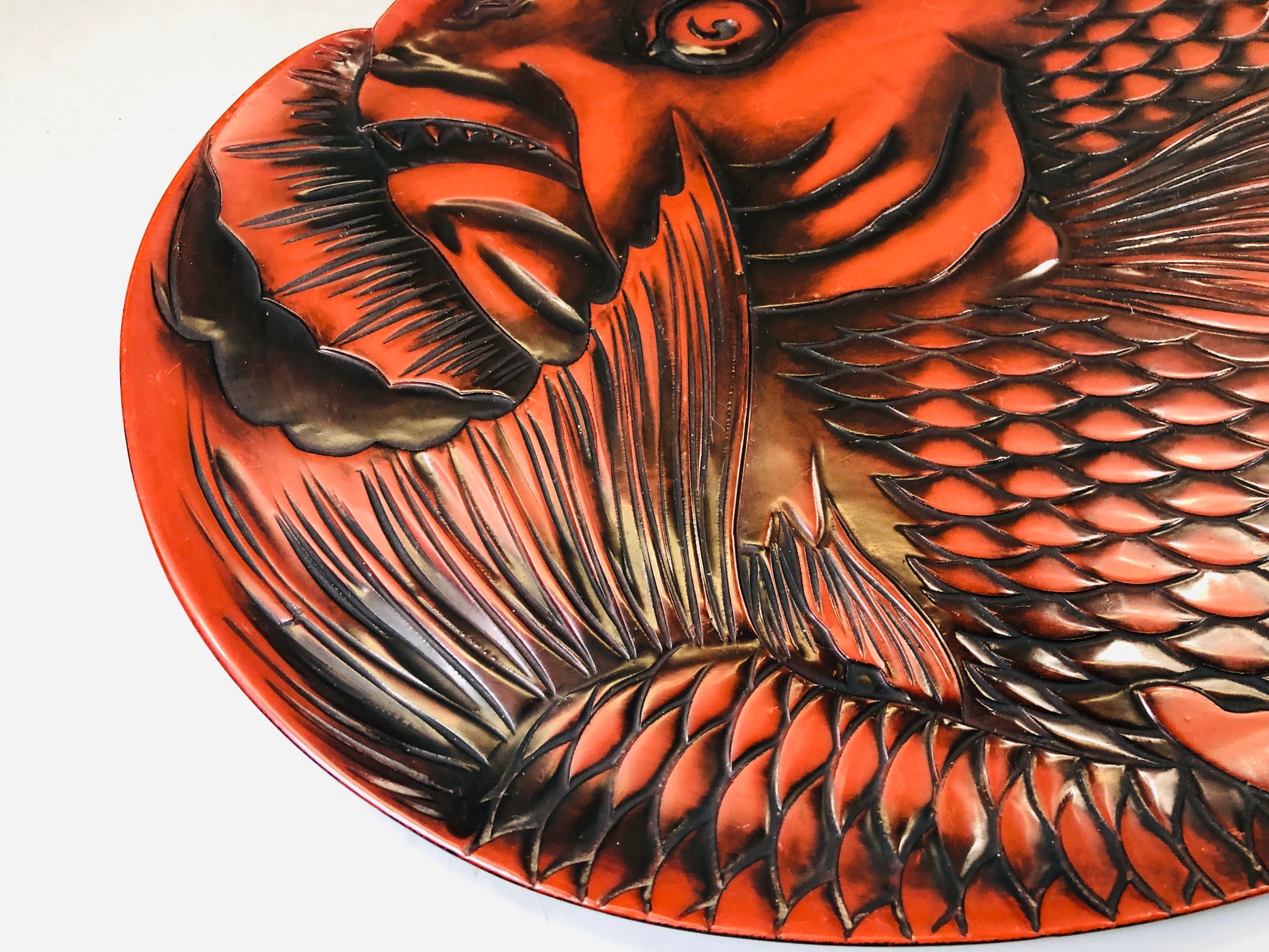The image features a detailed depiction of a fish on what appears to be a round or possibly oval platter or dish. The primary colors are a reddish-cinnamon-orange and black. The fish design is highly intricate, with noticeable black scales and black outlining the various features, including the face, eyes, mouth, and fins. The fish's face, under the tail, is prominently black, as are the areas between the scales, adding to the texture and depth. The background that is visible is orange. The image cuts off part of the dish, leaving the right edge and parts of the top not fully visible. Towards the middle of the image, there's a fin and the tail fin, curving in such a way that it gives the impression of the fish being wrapped around. Additional fins are visible towards the top right and middle top, with more scales decorating the bottom right and right side of the image, creating a circular, almost spiral-like effect.